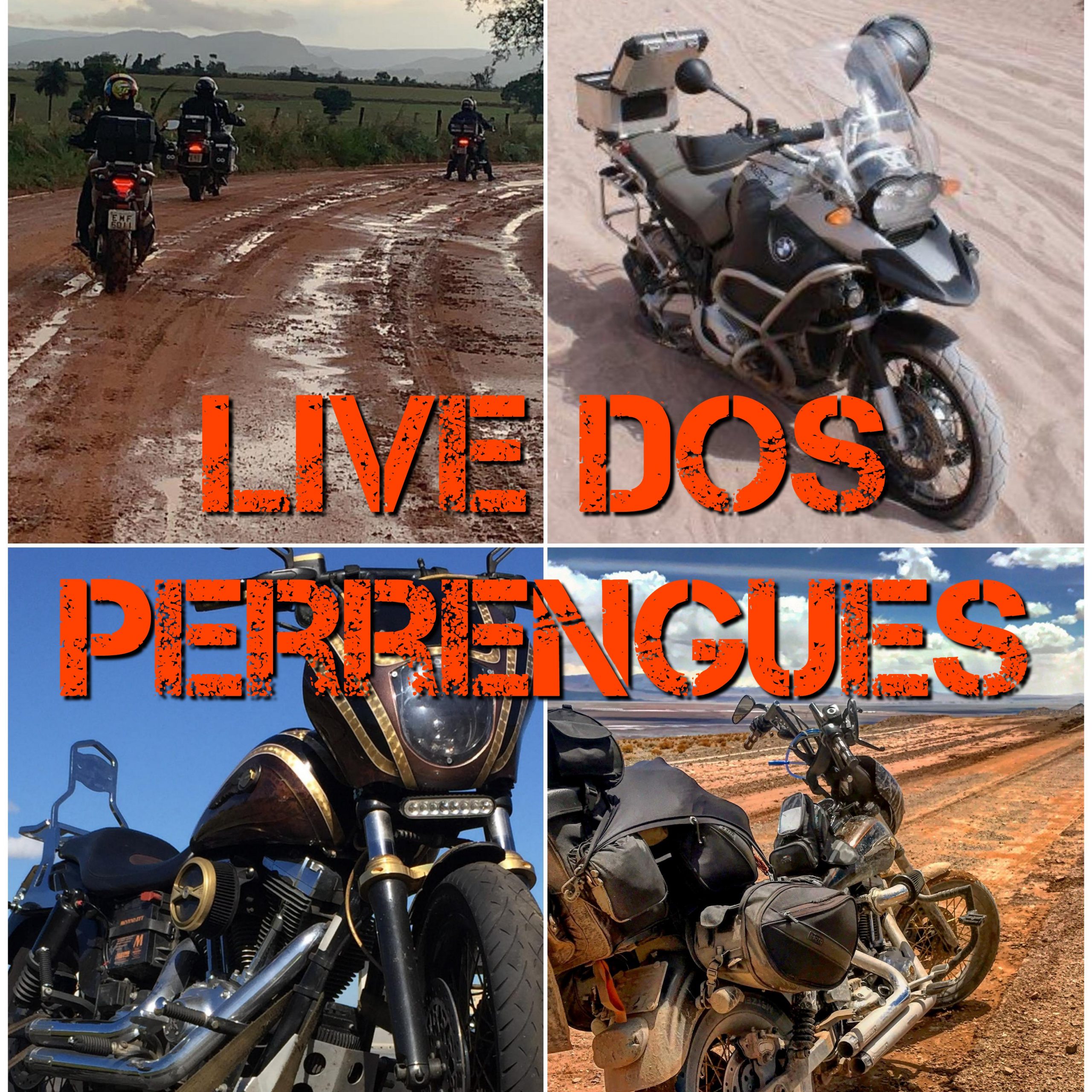The image is centered around a large, bold red font that reads "LiveDAS P-E-R-R-E-N-G-U-E-S," likely an advertisement for a motorcycle group. The layout is a single large square divided into four smaller squares by white vertical and horizontal lines. Each quadrant features a distinct motorcycle scene. The top left picture shows three riders navigating a muddy dirt road, set against a backdrop of open fields, trees, and distant mountains beneath a cloudy sky. The top right image captures a stationary bike parked on sand, equipped with an open container at the back and a helmet placed on the handlebar. In the bottom left section, a black and gold motorcycle is parked with the sky serving as the background. The bottom right image displays another motorcycle parked on a dirt road. The overall theme of the image is to showcase various motorcycles and scenes from rides, emphasizing a sense of adventure and versatility.